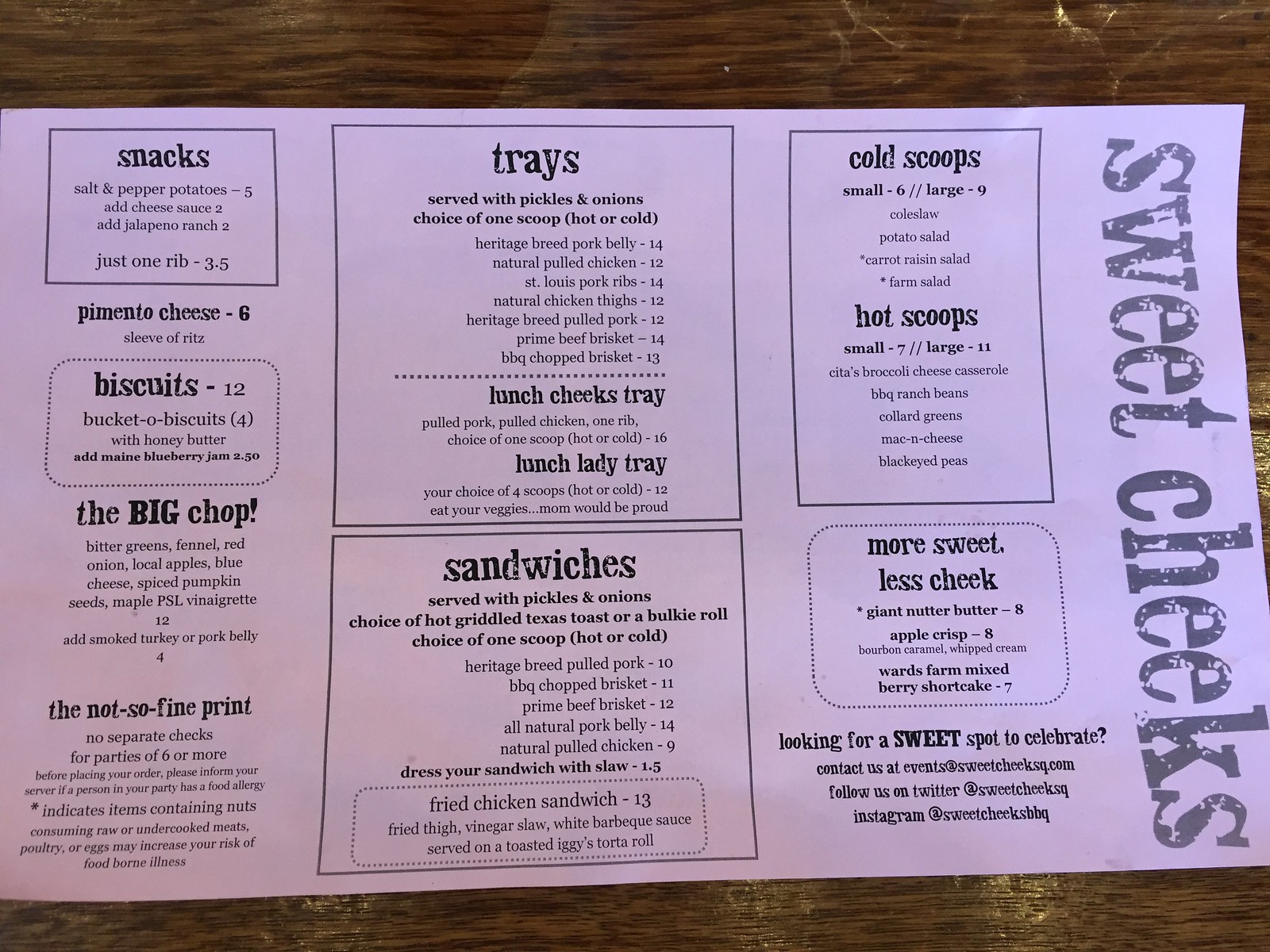This image showcases a pink menu laid out vertically on a brown, wooden-grain table. Down the right side, the heading "Sweet Cheeks" is prominently displayed. The content on the left-hand side begins with a section titled "Snacks," followed by a section labeled "Biscuits." Below these is a heading with bold lettering that reads "The Big Chop," and further down, "The Not So Fine Print."

In the middle of the menu are two boxes: the top box is titled "Trays" and lists options such as "Lunch Cheeks Trays" and "Lunch Lady Tray." The bottom box is labeled "Sandwiches" and includes options, with a specific mention of a "Fried Chicken Sandwich" at the very bottom.

To the right of these two boxes is another section titled "Cold Scoops and Hot Scoops." Below this, there's a phrase "More Sweet, Less Cheek," followed by a note indicating, "Looking for a sweet spot to celebrate? Contact us at this web address."

The entire menu, rich in detail and neatly organized, is photographed against a sturdy brown table, with the wood grain clearly visible, adding a warm, rustic touch to the overall presentation.